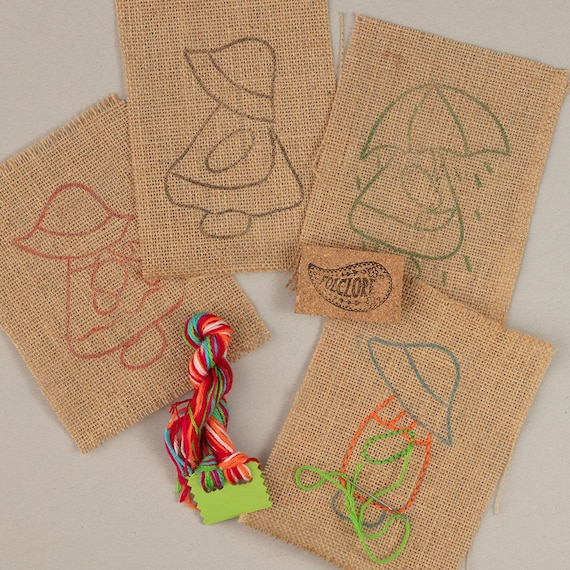The image showcases four embroidered burlap squares, each featuring printed stitching guidelines, positioned as if for a crafting project display. These small burlap pieces appear prepped for intricate embroidery designs, with one completed piece displaying colorful green and orange stitches that align with the visible printed templates on the other squares. The stitched design suggests a simplistic profile of a girl, possibly with a dress and arm-like ovals, evoking a basic, perhaps childlike, image reminiscent of characters like Paddington Bear. Accompanying the burlap squares is a bundle of yarn loops, likely intended for the embroidery, and a stamped piece of cork bearing the name "Folklore," indicating the brand or crafting kit name. The detailed setup suggests this could be intended for sale as handcrafted goods, possibly on platforms like Etsy.